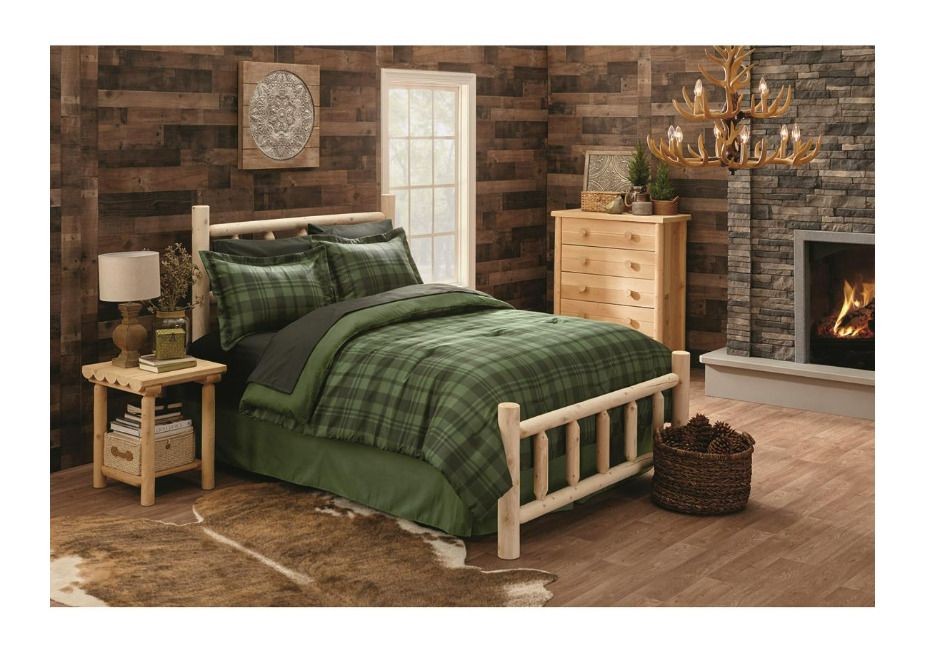This image portrays a cozy bedroom that exudes a rustic, cabin-like charm with both traditional and modern elements. Dominating the left side of the space is a warm-toned wooden wall, reminiscent of a cabin, complemented by horizontal wooden panels alternating in light and dark shades. Leaning toward the bed, there's a bearskin rug sprawled across the floor, adding a touch of wilderness. The wooden bed frame, with its headboard and footboard, supports a green, plaid-patterned bedspread accompanied by four pillows – a mix of green and black, harmonizing with the sheets underneath. 

Adjacent to the bed stands a wooden nightstand, organized with a lamp, a flower pot, and several books, with additional books stored in a box beneath it. Above the bed hangs a portrait, its details hinting at artistic nuances, and to the right of the bed is a large window allowing natural light to cascade into the room. A wooden dresser, topped with another portrait and some plant decor, adds to the functional elegance of the room. 

Hanging from the ceiling is a chandelier crafted to resemble elk or deer antlers, contributing to the room's rustic ambiance. In front of the bed, lies a basket full of large pine cones, enhancing the natural feel of the space. The room features a fireplace with a chimney covered in a brick-like pattern, which stands out on the right, adding both warmth and a focal point to the room. Altogether, the scene is rich in detail, evoking the tranquility and comfort of a sophisticated yet homey retreat.